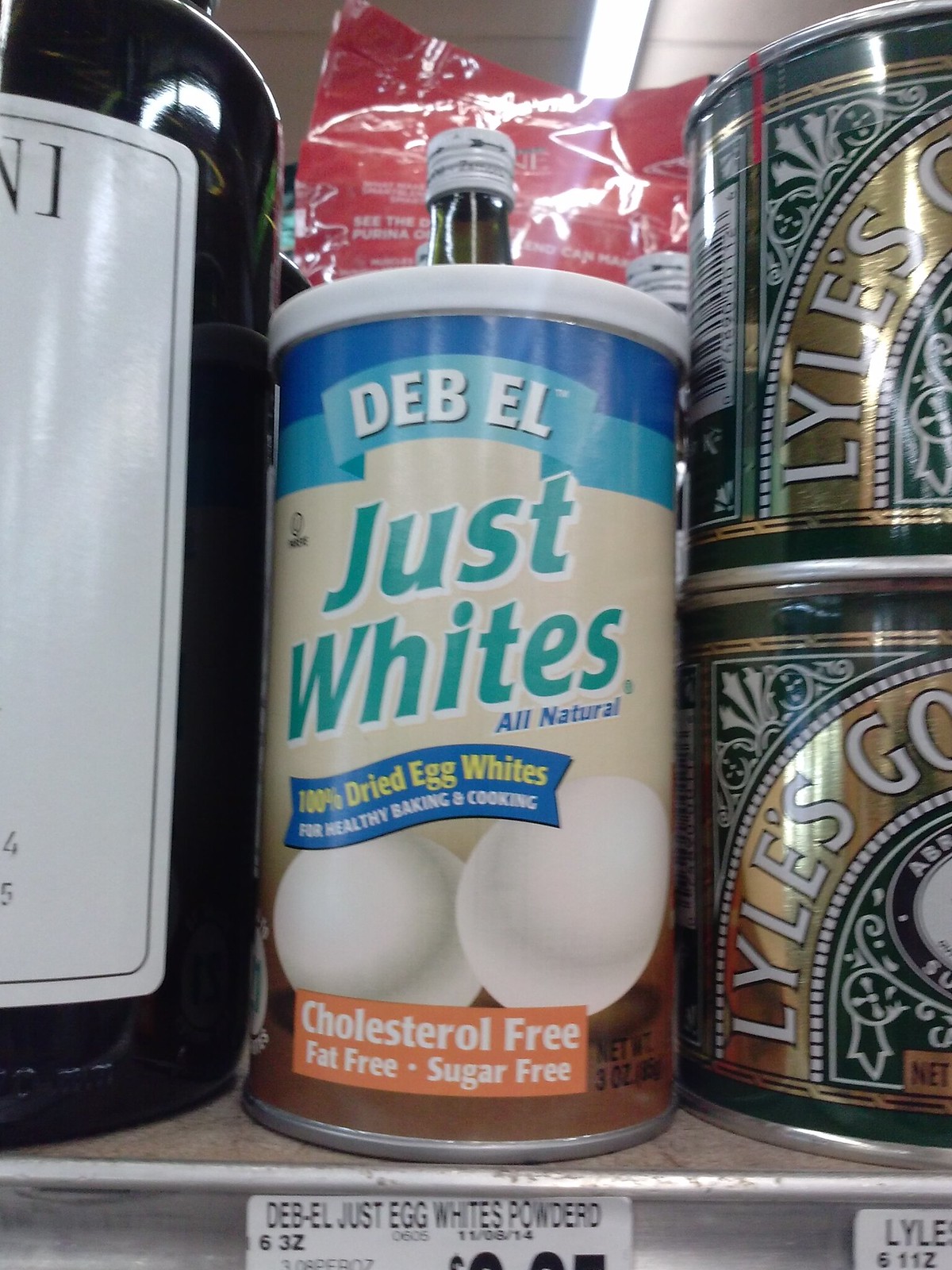This detailed close-up photograph captures a section of a store shelf displaying various food products, clearly denoted by the visible price tags. The central focus is a cylindrical tin of powdered egg whites by the brand Deb El, featuring a design that transitions from dark blue to cyan. The label, set on a cream and tan background, reads "Just Whites" in light blue and "All Natural 100% Dried Egg Whites" with a dark blue ribbon. It highlights that the product is cholesterol-free, fat-free, and sugar-free, with a suitable emphasis for healthy baking and cooking. The packaging also includes an image of two white eggs. To the right, partially visible, are tins of Lyle's Golden Syrup, identifiable by their green and gold design with partially obscured white embroidery that reads "G.O.". To the left, there is a tall, dark-colored bottle with a white label, possibly resembling a wine bottle. The shelf is metallic and light brown on the top, under fluorescent lighting, further indicating a retail environment.